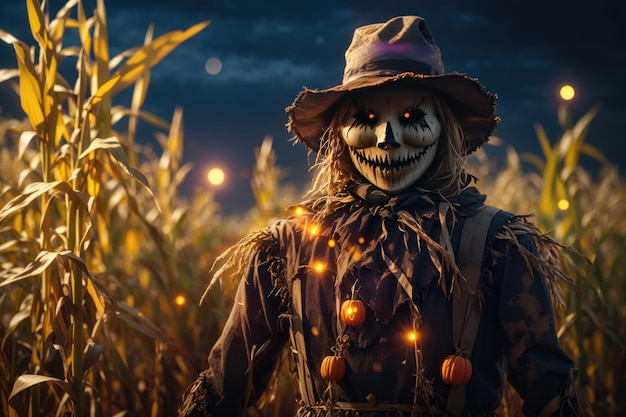The image is a digitally rendered scarecrow standing menacingly in a cornfield at night, exuding an eerie vibe reminiscent of a horror film. The scarecrow has a realistic, pale face with a jagged, stitched-like smile and glowing orange eyes under a tattered straw hat with a band. Its raggedy clothes, frayed at the edges, reveal straw poking out from the neckline and shoulders. A garland of tiny pumpkins, some glowing, decorates its chest. The background is a dark, stormy sky with a bright but small, mist-covered full moon, and dead corn stalks stretch out below. The scarecrow, visible from head to lower chest, faces the viewer directly, enhancing the unsettling atmosphere.